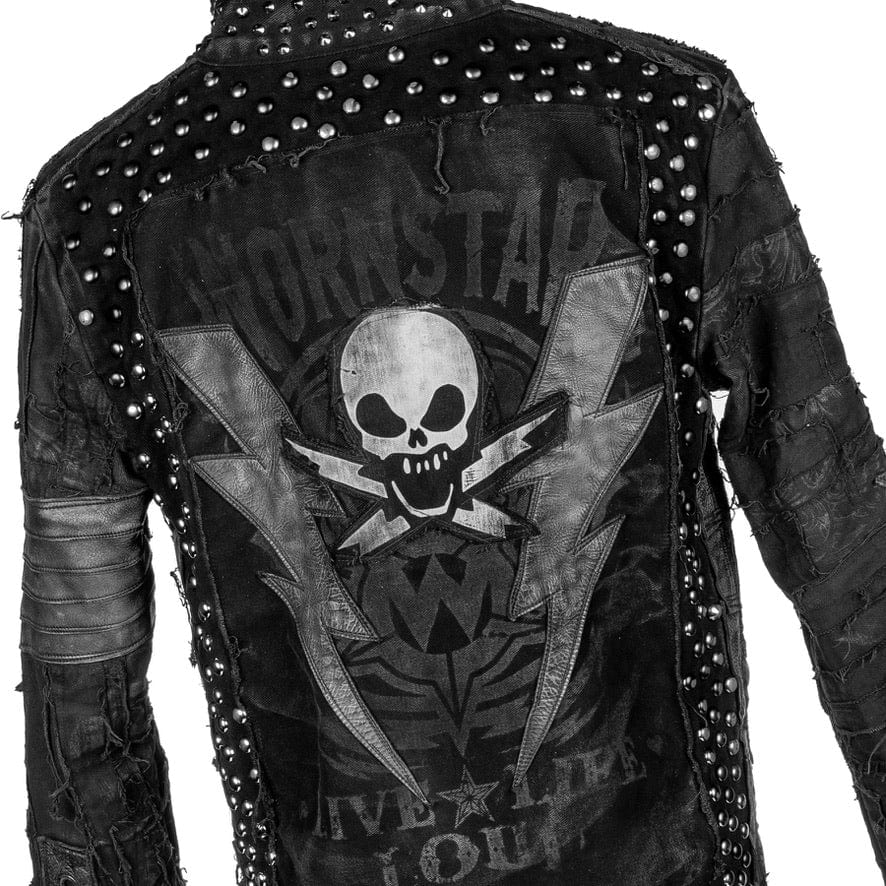The image displays the back of a high-end black leather jacket adorned with various intricate details. Centered on the back is a prominent, screaming skull with lightning bolts in place of crossbones, emphasizing a rebellious and bold design. Above the skull, the word "Hornstar" is inscribed, while below it, the phrase "Live Life Loud" is prominently displayed alongside a five-point star. Surrounding the skull are dull gray lightning bolts, further enhancing the edgy aesthetic. Metal studs or beads are meticulously lined along the shoulder and down the sides of the jacket, adding a rugged yet refined touch. Additionally, a circular patch featuring the letter "W" with four radiating points is situated below the skull, contributing to the jacket's detailed and complex appearance. The overall background of the image is white, providing a stark contrast that highlights the jacket’s design elements.